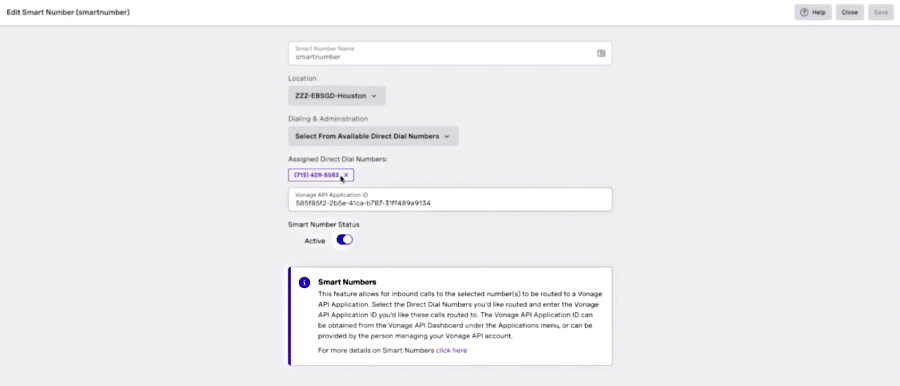**Descriptive Caption:**

This is a screenshot of a webpage, predominantly rectangular in shape, with greater width than height. The background is grey with a white bar running across the top. In the top left corner, the text "Edit Smart Number (Smart Number)" is displayed. On the right side of this bar, there are three buttons labeled "Help", "Close", and "Save". The "Save" button is greyed out, while "Help" and "Close" have a grey background with bold black lettering; notably, the "Help" button includes a question mark icon.

Centrally located on the page is a drop-down menu labeled "Smart Number Name", followed by a field titled "Smart Number". Below this, another dropdown, under the heading "Location", reads "ZZZ EBSGD Houston" against a grey backdrop. Further down, under the section "Dialing and Administration", there is a dropdown menu labeled "Select from Available Direct Dial Numbers". 

Below this, the text "Assign Direct Dial Number" precedes a phone number displayed in purple, 713-429-5582, with an arrow pointing to it. Further down, a lengthy authentication number is shown along with a white input bar.

At the bottom of the page, under the heading "Smart Number Status", there is a toggle switch set to "Active", highlighted in blue. Finally, towards the bottom, the section labeled "Smart Numbers" explains: "This feature allows for inbound calls to the selected numbers to be routed to a Vonage API application." Additional descriptive text follows below this explanation, but it is not fully visible in the screenshot.